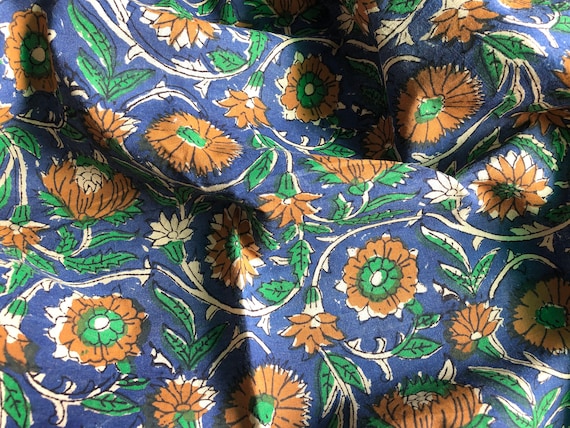The image displays a close-up view of a ruffled fabric featuring a vibrant dark blue background adorned with an intricate floral pattern. The main flowers are a distinctive burnt orange with an emerald green center. These flowers are scattered throughout the fabric, blooming from white vines that curl and weave across the design, accompanied by long, slender leaves. Some flowers have finely detailed petals, while others are somewhat less defined, with spikes or more rounded forms. Notably, there are areas where the color from the flowers bleeds slightly onto the blue background, creating white outlines in places. Smaller white flowers with green bases are also interspersed amidst the larger blooms. The overall pattern appears hand-painted and intentionally offset, lending a unique charm to the fabric. Shadows and light play across its ruffled surface, highlighting the vibrant and equally distributed floral design.